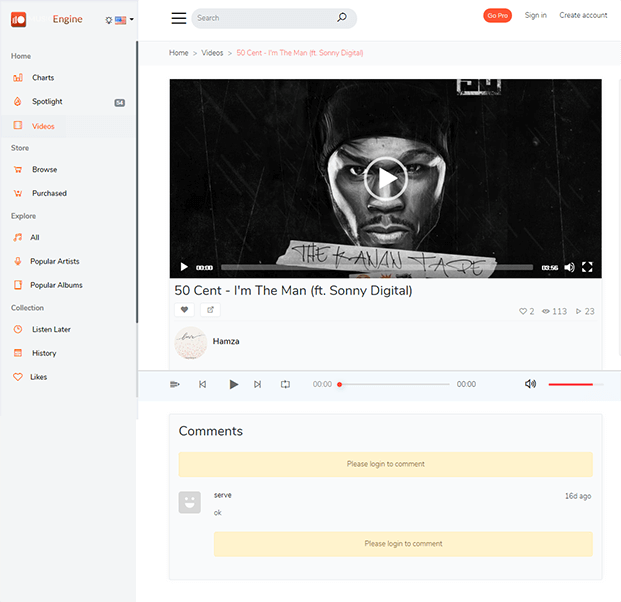The image showcases a detailed view of a web page with various sections and interactive elements. 

### Header and Side Navigation
- **Background**: Predominantly white with a vertical light gray section on the left.
- **Top Left Corner**: An orange square with a white circle in the center, featuring the word "Engine" in capitalized orange text. Adjacent icons include a location marker, an American flag with a downward arrow indicating more options, and the word "Home" in gray text.
- **Navigation Options**:
  - "Charts" with an adjacent orange logo
  - "Spotlight" with an adjacent orange logo
  - "Videos" in orange text accompanied by a filmstrip logo
  - "Store" section featuring an orange shopping cart and "Browse" in black text, followed by an icon of a shopping cart with three squares labeled "Purchase"
  - "Explore" section with the following:
    - Musical note labeled "All"
    - Microphone labeled "Popular Artists"
    - Square object labeled "Popular Albums"
  - "Collection" section in gray, including:
    - Circular orange object labeled "Listen Later"
    - Orange square labeled "History"
    - Orange heart labeled "Likes" 

### Main Content
- **Upper Center**: Three stacked horizontal lines and a gray search bar labeled "Search" with a magnifying glass icon.
- **Right Section**:
  - Orange tab labeled "GoPro"
  - Gray tabs labeled "Sign In" and "Create Account"
  
### Video Section
- **Breadcrumb Navigation**: "Home" > "Video" > "50 Cent - I'm the Man (featuring Sonny Digital)"
- **Thumbnail**:
  - Black background featuring 50 Cent’s face wearing a black hat
  - White play button circle
  - Bottom text in white on a tape-like strip: "The Canon Tape"
- **Video Controls**:
  - White play triangle, time indicator, gray status bar, and a white speaker icon
  - Full screen icon
  - Gray title: "50 Cent - I'm the Man (featuring Sonny Digital)"
  - Gray heart icon
  - White marker (text unreadable)
  - Far right: gray heart (number 2), play icon (number 113), and avatar with the name "Hamza"

### Player Controls:
- Blue bar with several icons: Rewind, Play, Fast Forward, Looped Arrow
- Time bar with orange dot
- Right side: Speaker icon with an orange volume line

### Comment Section:
- **Light Blue Square**: "Comments" in black text at the upper left corner
- **Yellow Bar**: "Please log in to comment" in black text at the center
- **Comments**:
  - User "Serve" with gray square avatar featuring a smiley face, commented "okay" 16 days ago
  - Another time bar with "Please log in to comment"

This comprehensive caption describes the detailed layout and interactive elements of the web page, offering a clear picture of the user interface and content.